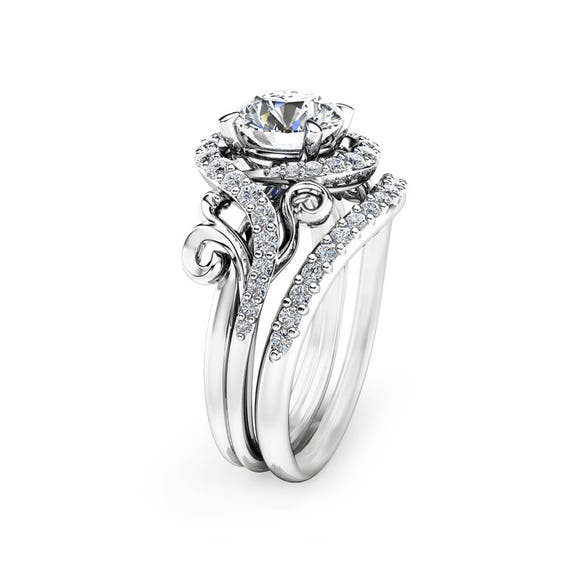The image showcases a stunning ring set composed of three bands. The set includes both an engagement ring and a wedding band, viewed from the side to highlight the intricacies of the design. The central band features a prominent, solitary diamond encircled by a diamond halo, adding to its brilliance. This central band is adorned with small diamonds that extend halfway up and curve around the top, creating a visual halo effect around the large diamond. The band on the right is encrusted with small diamonds on its upper surface, while the band on the left appears simpler and undecorated. The bands are designed to fit seamlessly together, forming a cohesive and elegant set. The entire ring set is presented against a plain white background, accentuating its intricate details and sparkling diamonds without any distractions.